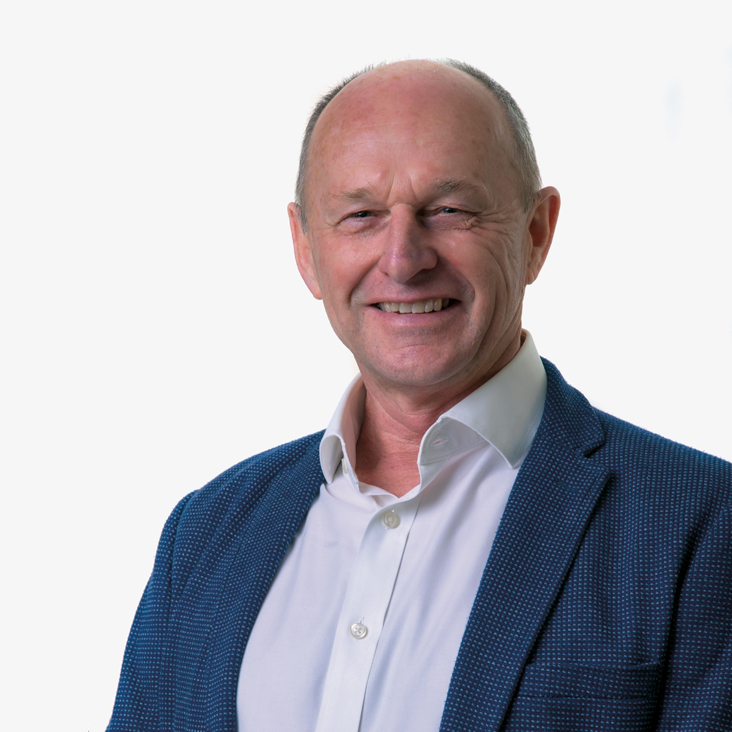This photograph portrays an older white gentleman, likely in his late 50s to early 60s, standing against a white background. He has a receding hairline with short, salt-and-pepper hair on the sides and back of his head. His face is clean-shaven, featuring visible laugh lines around his mouth and eyes, suggesting a pleasant demeanor. He is smiling warmly with slightly squinted eyes, displaying nice, though slightly off-white, teeth. 

He is dressed in a crisp white button-up shirt with the top button undone, paired with a dark blue, tweed-like blazer adorned with tiny light blue and dark blue checks, creating a subtle, sophisticated pattern. The blazer also features a pocket on the left breast area. The photograph is cropped mid-chest, focusing primarily on his upper body, and appears to be taken for a professional profile, such as a LinkedIn picture. His complexion is clear, with a slight red tint, and the entire scene is neatly arranged, emphasizing his approachable yet professional appearance.